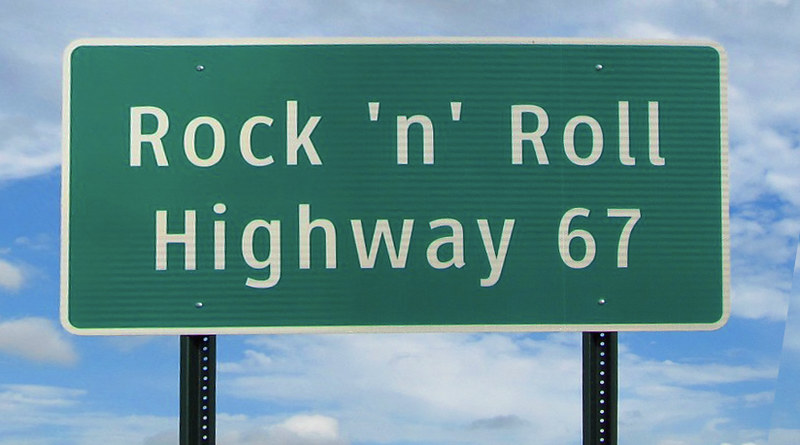The image features a rectangular green roadway sign with a white border, oriented horizontally. The sign prominently displays the text "Rock 'N' Roll Highway 67" in bold white characters. It is mounted on two nearly black steel posts with a distinctive humped metal shape and flanges at the bottom. Four silver fasteners are visible, securing the sign to the posts. The backdrop reveals a bright blue, partly cloudy sky, adding a vivid contrast to the scene.